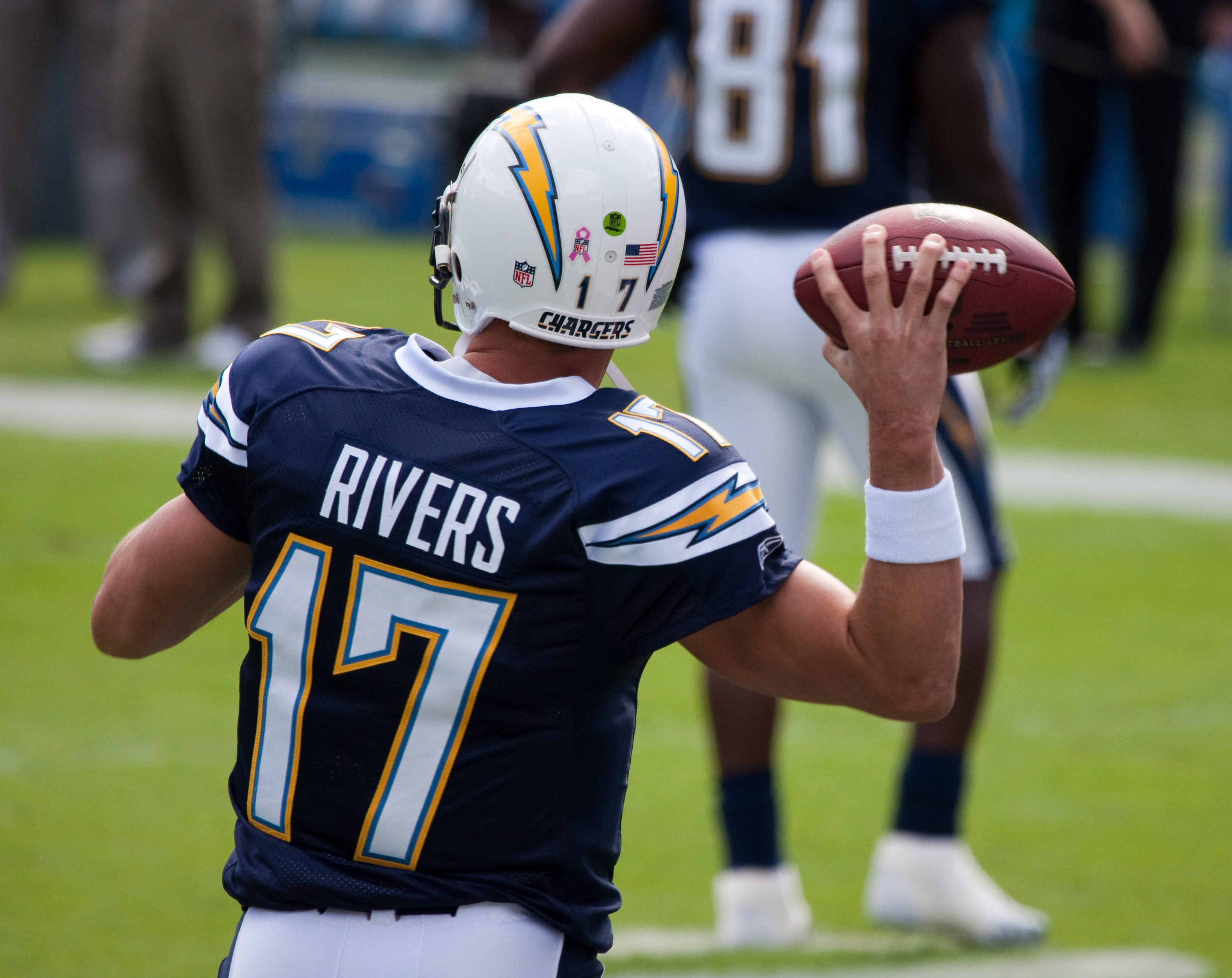In this photograph taken outdoors, we see NFL quarterback Philip Rivers preparing to throw a football. Captured from behind, Rivers is distinguishable by his blue jersey with "Rivers 17" emblazoned in white lettering, bordered in blue and yellow. His jersey is accented with yellow lightning bolts on the shoulders. Rivers is in mid-throw, his right arm pulled back, and he wears a white helmet adorned with blue and yellow lightning bolts, an American flag, the NFL logo, a pink breast cancer ribbon, and the word "Chargers." In the background, blurred figures populate the field and sidelines, including another player wearing the number 81 in a similar uniform. This image captures the essence of action on the field, likely during a game.